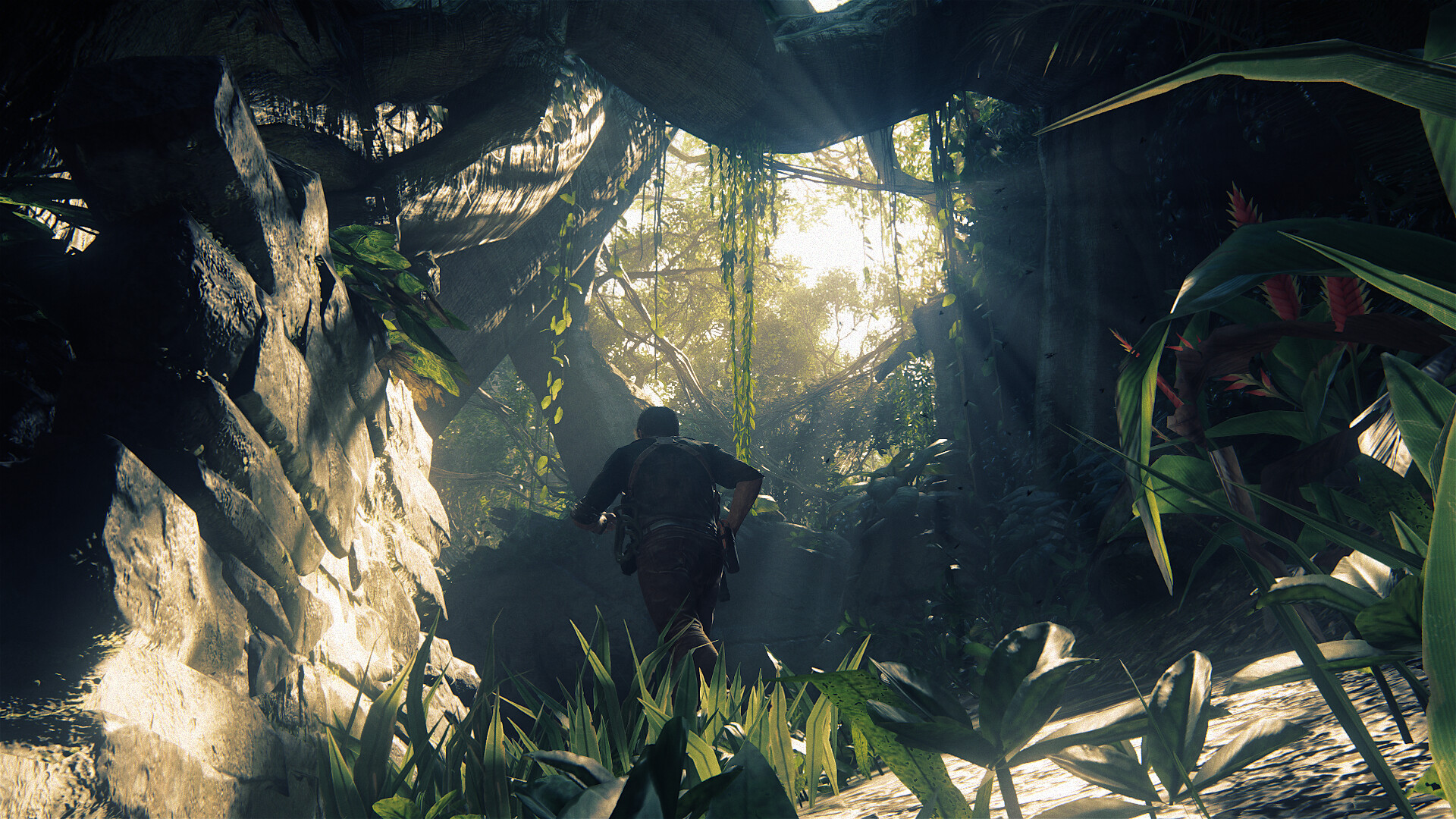The image depicts a highly realistic, possibly video game-inspired scene, capturing a man—who bears a resemblance to Nathan Drake from the Uncharted series—running through a dense, jungle-like forest. The orientation of the image is landscape, showcasing the man's back as he moves to the left side of the frame. He wears practical hiking attire, including brown pants, a dark-colored shirt with sleeves rolled up to his elbows, and a harness criss-crossing his upper back that seems to hold pouches on either side. He also appears to be holding a gun.

To the left of the man, there is a prominent outcrop of rocks with sun rays illuminating its surface. The ground beneath him is a mixture of dirt and broad-leaved tropical plants, with some areas gleaming in the sunlight penetrating the forest canopy. On the right side of the image, the scene descends into shade, where tall trees with visible trunks and long, dangling vines create a dense backdrop. Among the greenery, an orangey-red flower with yellow spikes stands out. The overall atmosphere is enhanced by beams of sunlight streaming through the trees, adding a sense of depth and adventure to the scene.